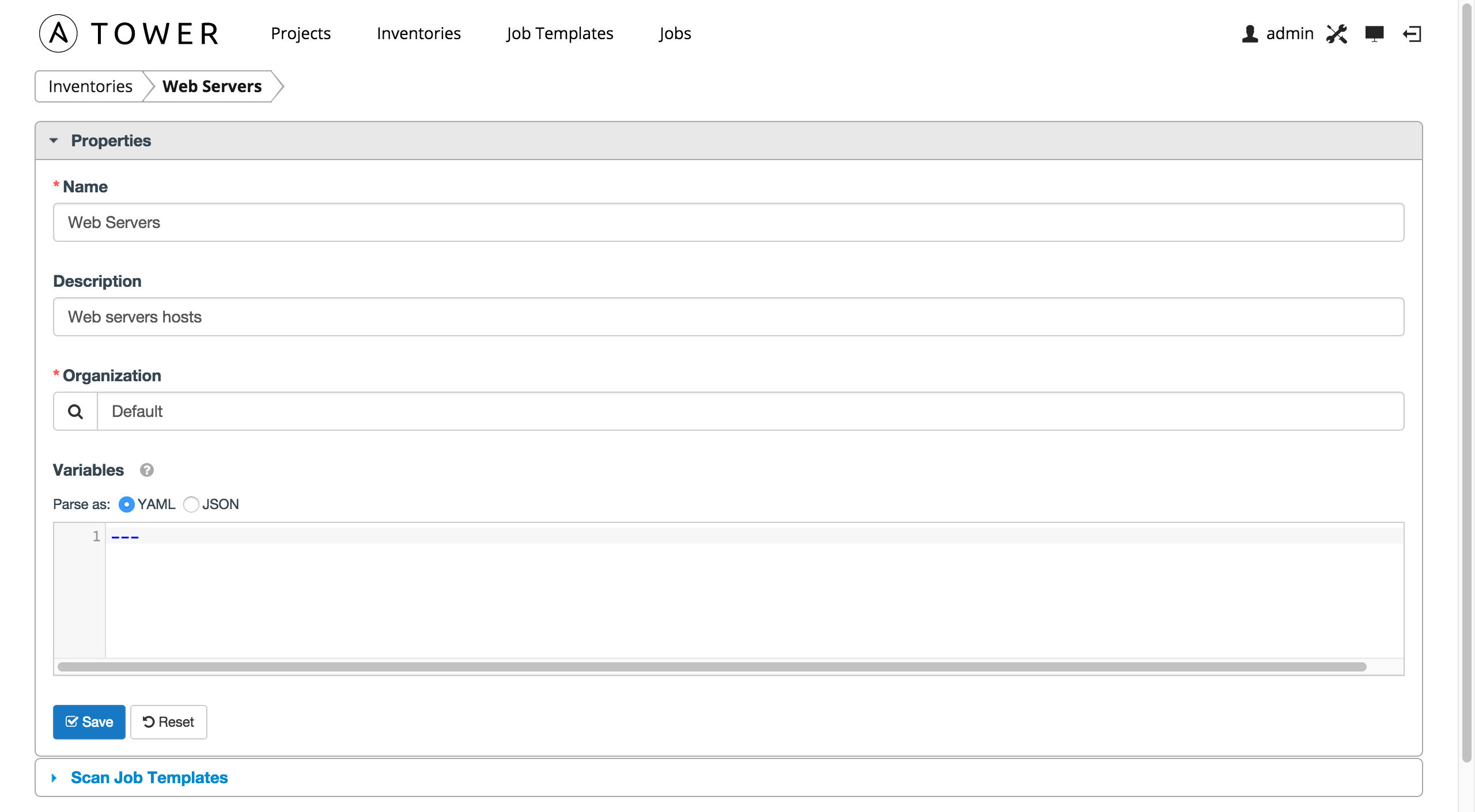The image is a detailed screenshot with a solid white background featuring elements in black, gray, and blue. In the upper left corner, a logo consisting of a circle with a small black flag is displayed, followed by the word "Tower" positioned to its right. Beneath the logo, a horizontal navigation menu is visible displaying the options: "Projects," "Inventories," "Job Templates," and "Jobs."

In the upper right corner of the screenshot, there is an icon representing a head and shoulders silhouette labeled "Admin," next to an image icon of a computer monitor.

On the left side of the screenshot, a light gray vertical sidebar is present, containing the sections "Inventories" and "Web Servers." Below this, the word "Properties" appears on a light gray banner. Directly underneath this banner, on a white background, there is a red asterisk next to the label "Name," followed by the text "Web Servers." 

Proceeding down the image, a section labeled "Description" features a box containing the text "Web Servers Hosts." Further down, the label "Organization" is displayed with a search box next to it containing the text "Default." Finally, the terms "Variables," "YAML," and "JSON" are listed at the bottom of the image.